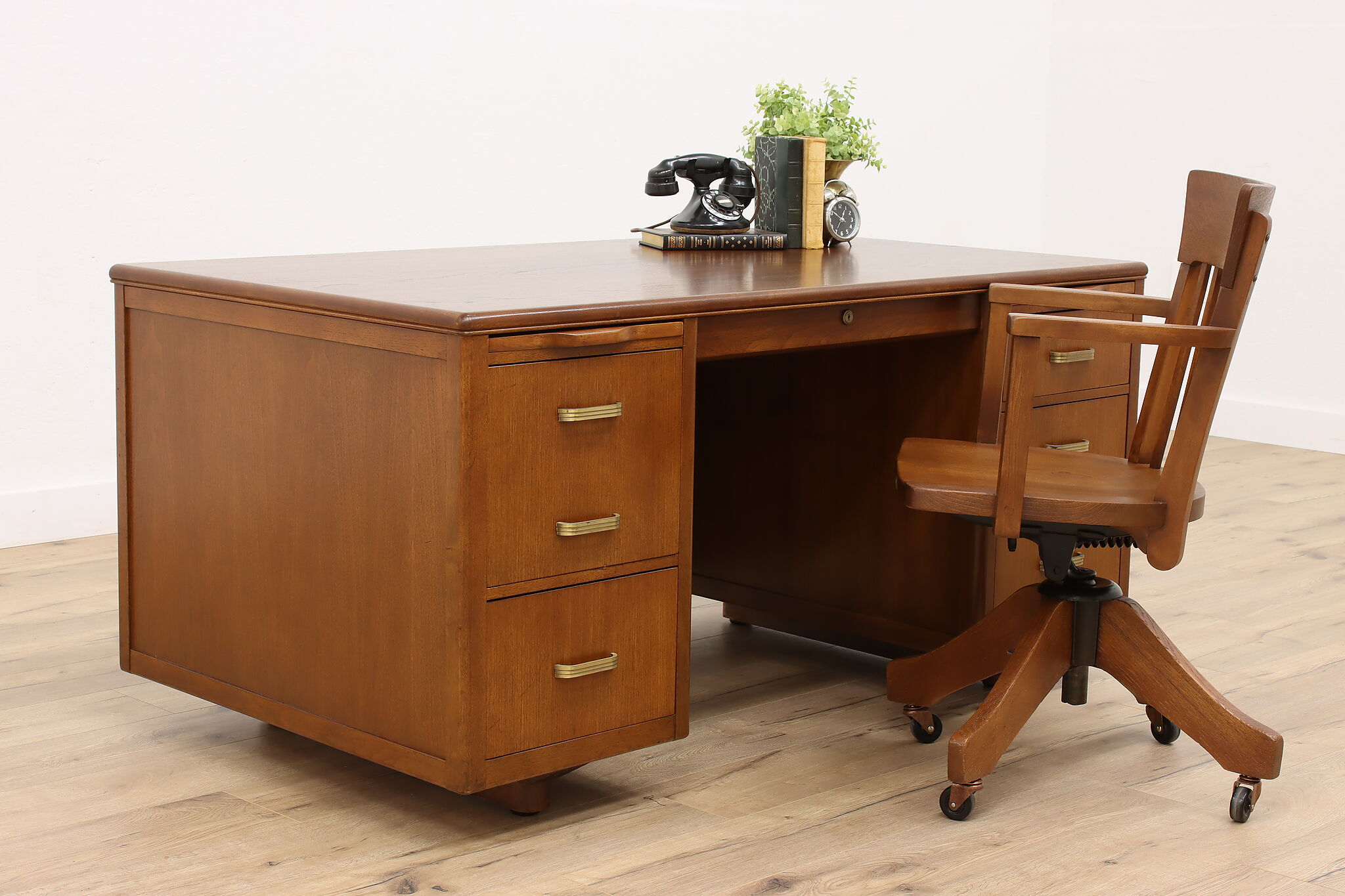This image captures a vintage wooden desk in what appears to be a minimalist room with plain white walls and light brown hardwood flooring. The medium-colored wooden desk, possibly dating from the 1930s to 1970s, features a symmetrical design with pull-out drawers on both sides. On the left, there are two drawers—a single-handled one at the bottom and a double-handled, taller drawer at the top. In contrast, the right side features the reverse: a double-handled drawer at the bottom and a single-handled one at the top. The middle has a thin, wide drawer with a round pull-out knob. The desk surface holds an arrangement of items: an old black telephone on top of a book in the upper right corner, a standing book, a brown planter with green leaves, and a small silver and black clock positioned in front of the planter. In front of the desk is a matching wooden swivel chair with four wheels, designed to easily slide under the desk and rotate as needed. The handles on the drawers vary in color, predominantly light golden but also include brown, black, green, tan, and white shades. This photo seems to be taken in a quiet indoor setting, perhaps a home office or a display room.